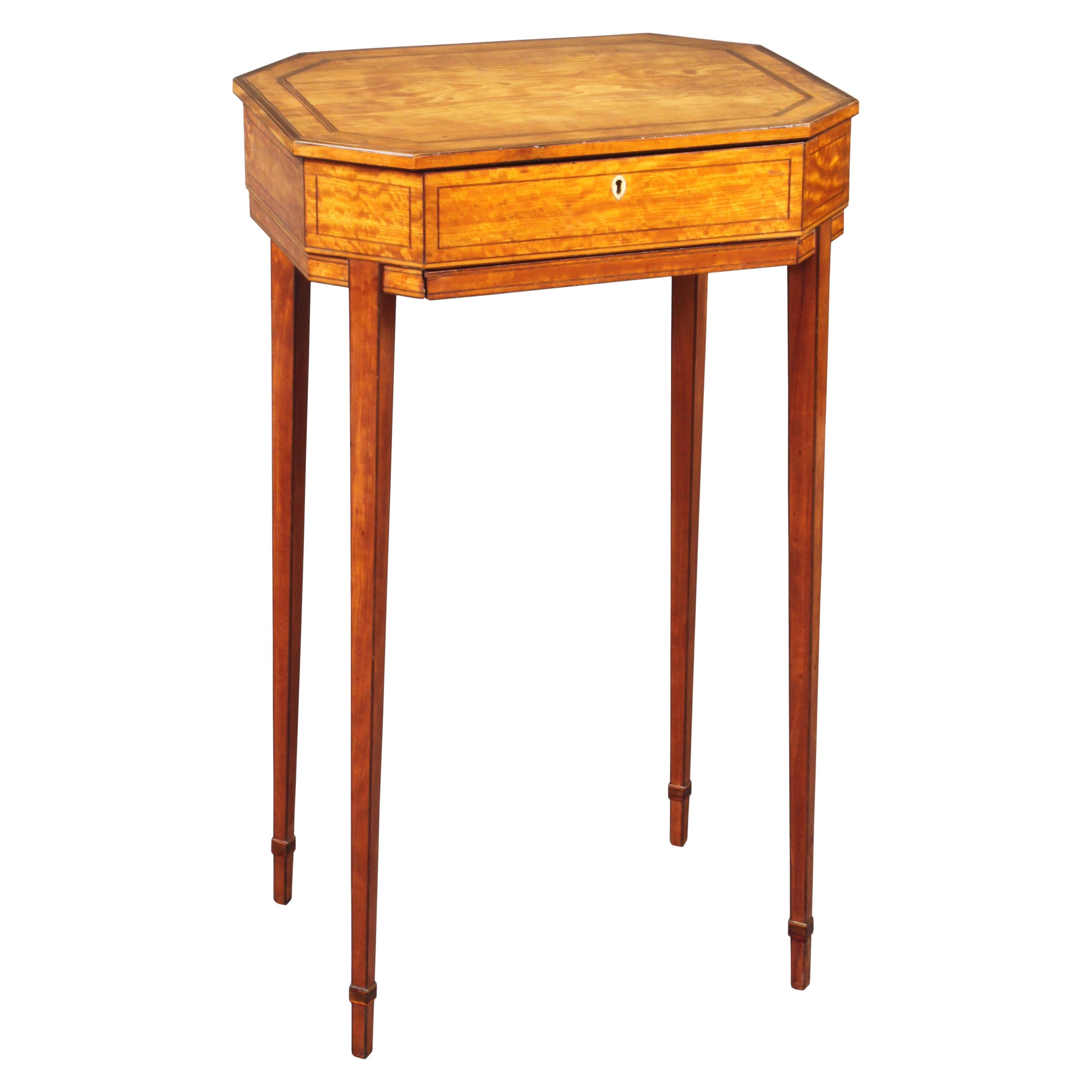In the image, there is a small, antique inn table crafted from walnut brown wood. The table features long, slender legs that taper to even smaller points and have decorative notches. The legs are a darker walnut color compared to the top. The tabletop itself is distinct with an intricate grooved pattern and an octagonal border inset about an inch from the edges, presenting a darker brown contrast. Additionally, the table includes a single drawer with a goldish-colored metal keyhole, indicating that it can be securely locked. The table, overall, exudes a rustic charm with its detailed craftsmanship and varying shades of walnut brown wood.